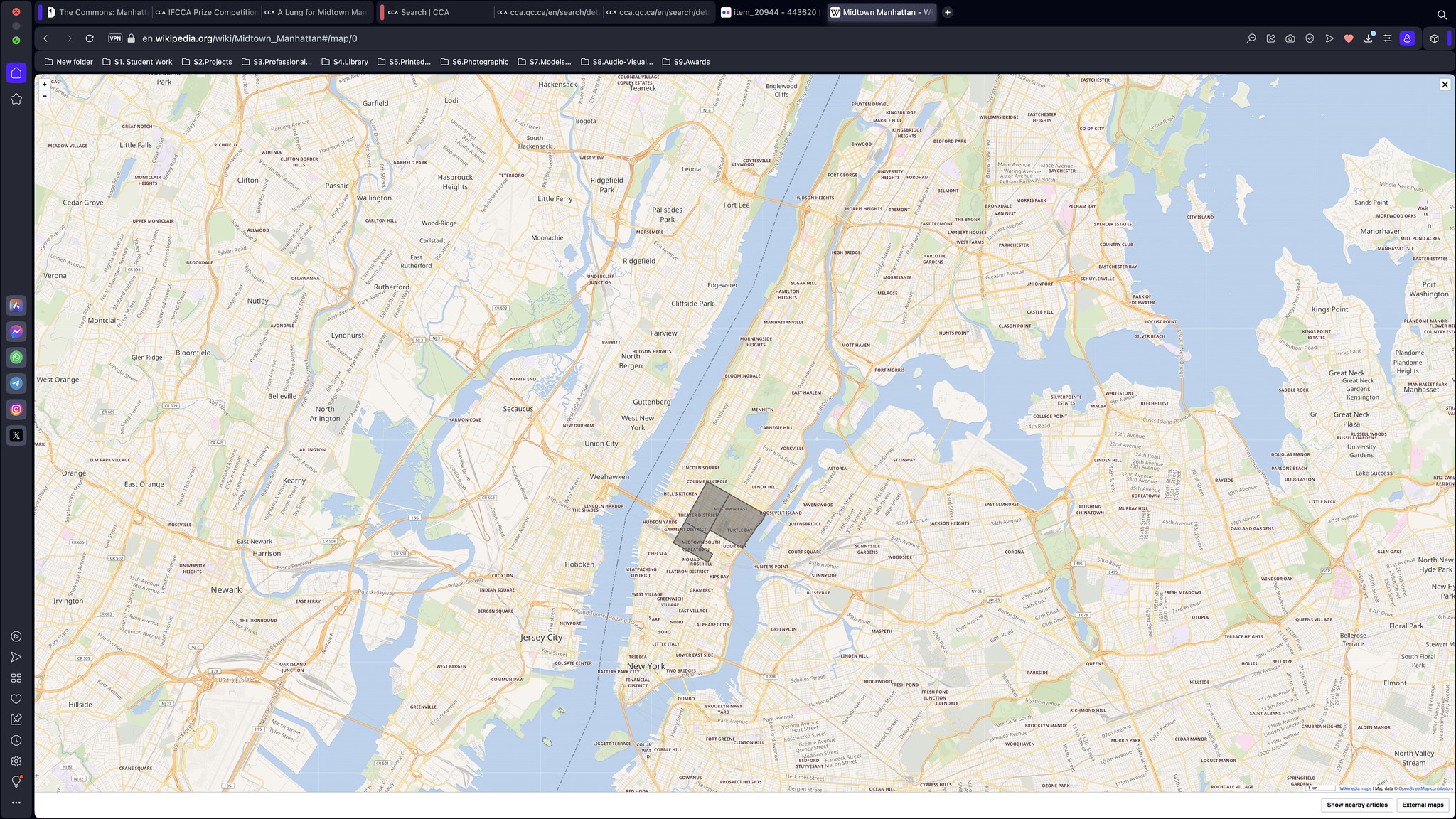The image is a detailed close-up of a city or state map, resembling the view from Google Maps. It features beige-colored landmasses surrounded by blue water bodies. The primary landmass dominates the left side, with the image cutting off diagonally from the top right to the bottom left. There is a smaller island-like feature situated between this main area and another landmass in the bottom right corner. The map is annotated with numerous names, though the text is too small to be legible. It also displays various colored markers and lines, including green spots and red-orange lines, indicating different types of information or routes. The map is shown within a dark-themed browser window, complete with visible tabs, an address bar, bookmarks, and a left-hand sidebar featuring different icons and menu options.